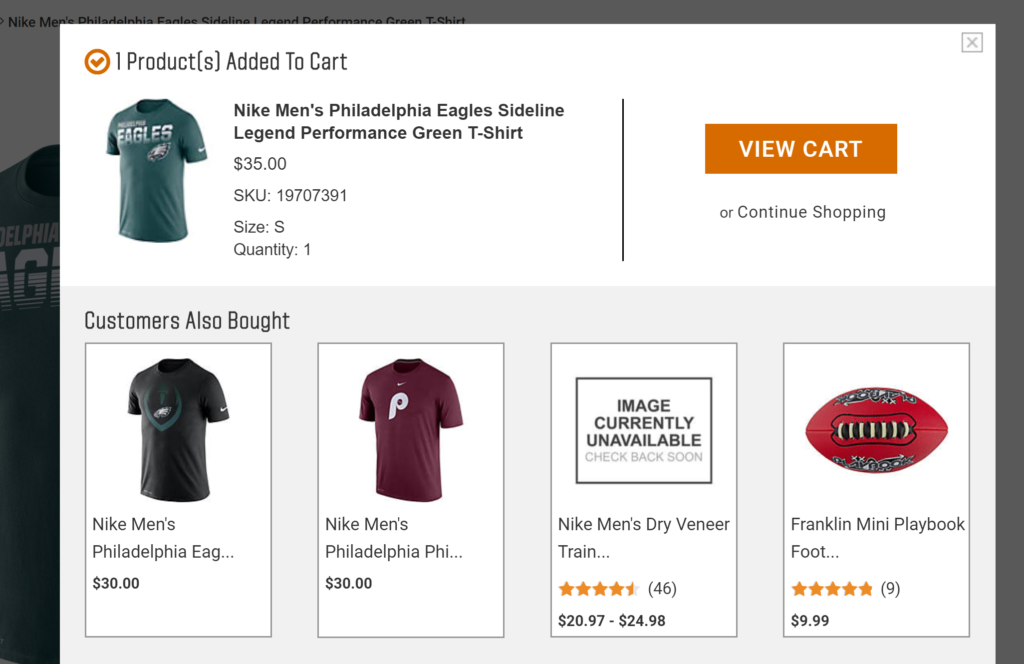This image depicts a screenshot from a sports apparel website, likely taken on a computer. The primary focus is a white rectangular notification at the top of the page indicating that one product has been added to the shopping cart. This message is highlighted by an orange checkmark within an orange circle.

The product added is a "Nike Men's Philadelphia Eagles Sideline Legend Performance Green T-Shirt," displayed in bold black font. Under this heading, the details include a price of $35, with an SKU of "19707391," size "S," and quantity "1." The green t-shirt, visible on the screen, features the word "Eagles" prominently and is designed for men based on the large sizing indicated.

To the right of the central product image, an orange button labeled "VIEW CART" appears in white capital letters. Below this button, another option in black text encourages users to "CONTINUE SHOPPING."

Further down, there is a gray box titled "CUSTOMERS ALSO BOUGHT" in black text. Inside this box are four vertically arranged white rectangles with thin black outlines displaying additional product recommendations. These include:

1. A "Nike Men's Philadelphia Eagles T-Shirt" priced at $30.
2. A "Nike Men's Philadelphia Phillies T-Shirt" also priced at $30.
3. A "Nike Men's Drive Into Your Training" t-shirt with prices ranging from $20.97 to $24.98 (text truncated as "Nike Men's Drive Into Your Train...").
4. A "Franklin Mini Playbook Football" priced at $9.99.

Each recommendation shows a small image and details of the respective products.